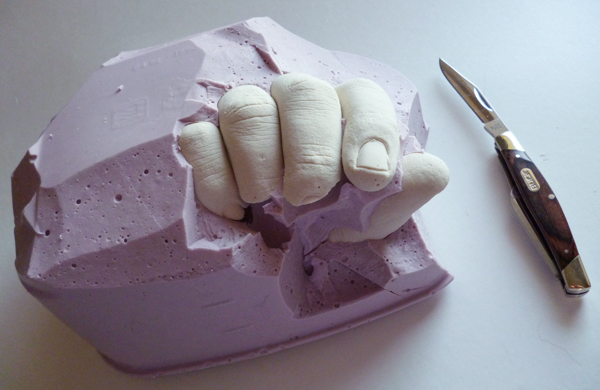On a white table, there is a molding of lavender-colored plaster, partially broken away to reveal the form of a right hand. The hand is molded in a slightly curled position, with four fingers distinct and the thumb visible on the right side. Next to the plaster hand rests an open, black pocket knife with silver tips, presumably used to scrape away the plaster. The scene, set against a very light blue background, captures the surreal and meticulous process of unveiling the encased hand from within the dried plaster.